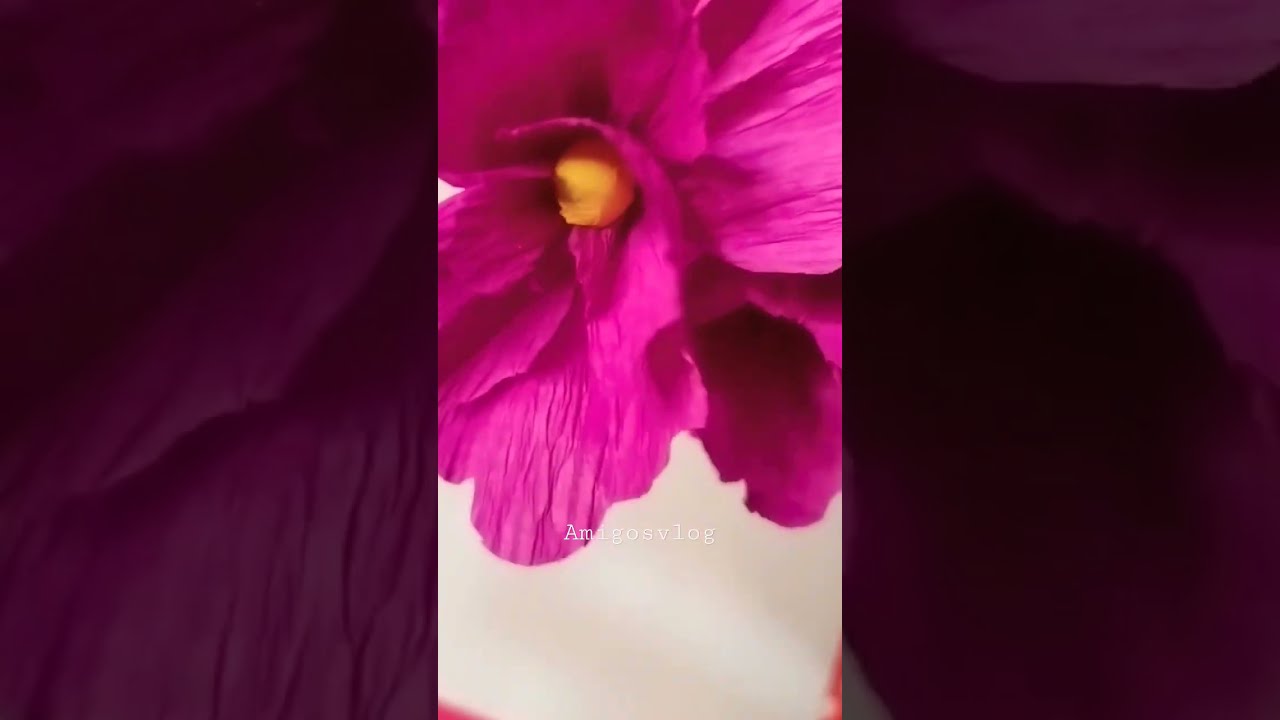The image is a wide horizontal rectangle comprising three tall vertical photographs. In the middle, there is a prominent, tall rectangular photograph of a bright maroon flower, its large and somewhat crinkly petals extending beyond the frame's top and sides. The center of this flower features a yellow, sphere-shaped object positioned towards the top left corner. The background of the middle image, visible only at the bottom, is a light beige. To the left and right of this central photograph are slightly wider vertical images showcasing close-ups of the central flower but shaded much darker, creating a stark contrast. The petals of the flower in the central image are a vibrant purplish-pink. At the bottom of the middle image, in thin white text, reads "Amigos Vlog," partially obscured by the ovary petal. The overall appearance of the composition suggests it may be a still shot from a video.